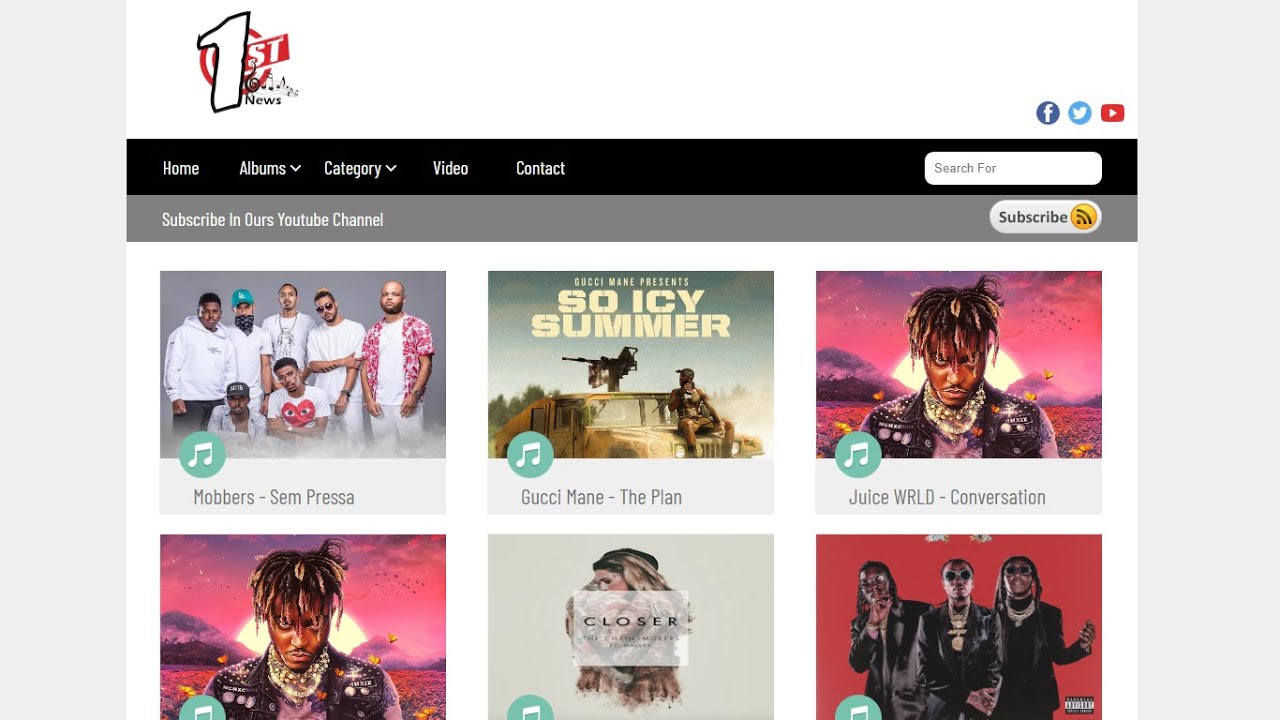The image is a screenshot of a hip-hop or R&B oriented music website. At the top left corner, the site features a logo for "First News," characterized by an italic font with an "ST" on a red field, encircled by a red target. On the far right side of the header, social media icons for Facebook, Twitter, and YouTube are prominently displayed.

Below this header is a black navigation bar containing menu options: Home, Albums, Category, Video, Contact, and a Search field on the far right. Immediately under the navigation bar, there is a gray line with text prompting users to subscribe to their YouTube channel, along with a subscribe button.

The main content showcases a grid of music-related thumbnails, organized in three columns across and two rows down, with additional content possibly visible if scrolled. The thumbnails appear to highlight album covers or promotional images of artists. 

- The first thumbnail in the top left features seven men against a gray background with the title "Mobster, Sampresa."
- Adjacent to this, the next thumbnail shows "Gucci Mane, The Plan" with a visual of a Humvee mounted with a machine gun.
- Another thumbnail for "Juice WRLD, Conversation" depicts an artist with dreads looking forward, set against a pink background featuring a setting sun.

On the second row:
- The thumbnail on the left, possibly repeated, is joined on the right by an image of a man and a woman embracing.
- Further to the right, there are three men wearing large sunglasses, though their identity is not immediately recalled.

A light green circle with a musical note is slightly visible in the bottom left of the image, suggesting an interactive or dynamic element. Overall, the screenshot appears to be a detailed mock-up rather than a live, functional website.